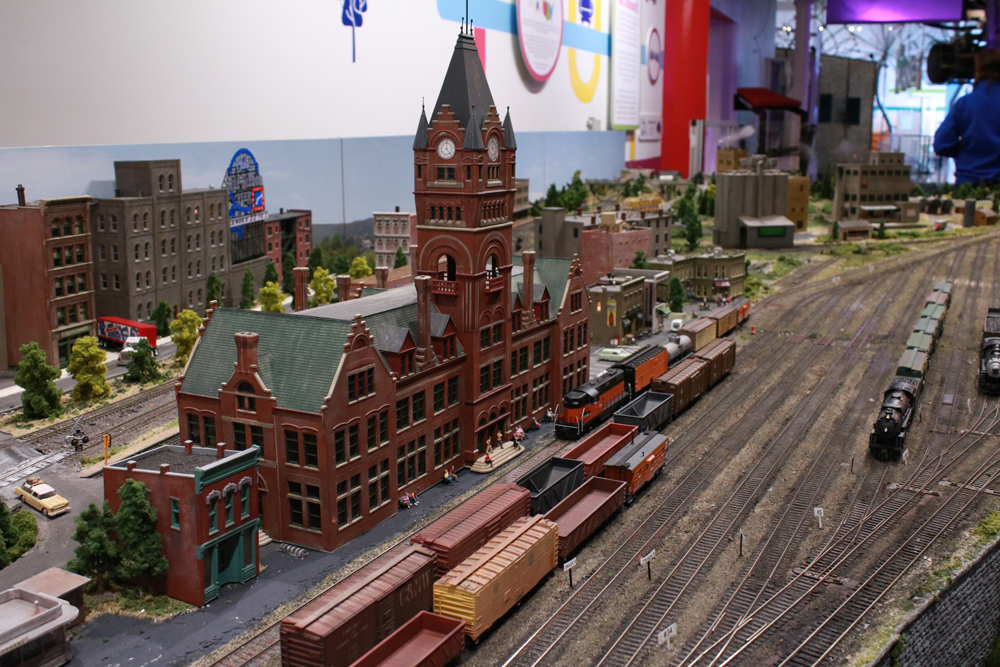The photograph captures an elaborate and meticulously detailed model train set, prominently featuring a network of train tracks and a variety of train cars including boxcars, a red train, and a black train approaching from the distance. At the center of the scene is a model of a city with interconnected buildings, ranging from brick structures to high-rise towers. Notably, a tall clock tower with small figurines of people at its base stands to the left of the image, next to a red train that seems to be at a train station. Additional buildings and structures, such as parking garages and possibly a college or park area, extend into the background, creating a sense of depth. Model cars and trees line the streets, adding to the realism of the cityscape. In the backdrop, a person in a blue jacket appears to be photographing or observing the model, enhancing the sense that this could be a museum exhibit. The overall scene is vibrant and bustling with miniature life, capturing the complexity and intricate craftsmanship of the model train set and its surrounding cityscape.